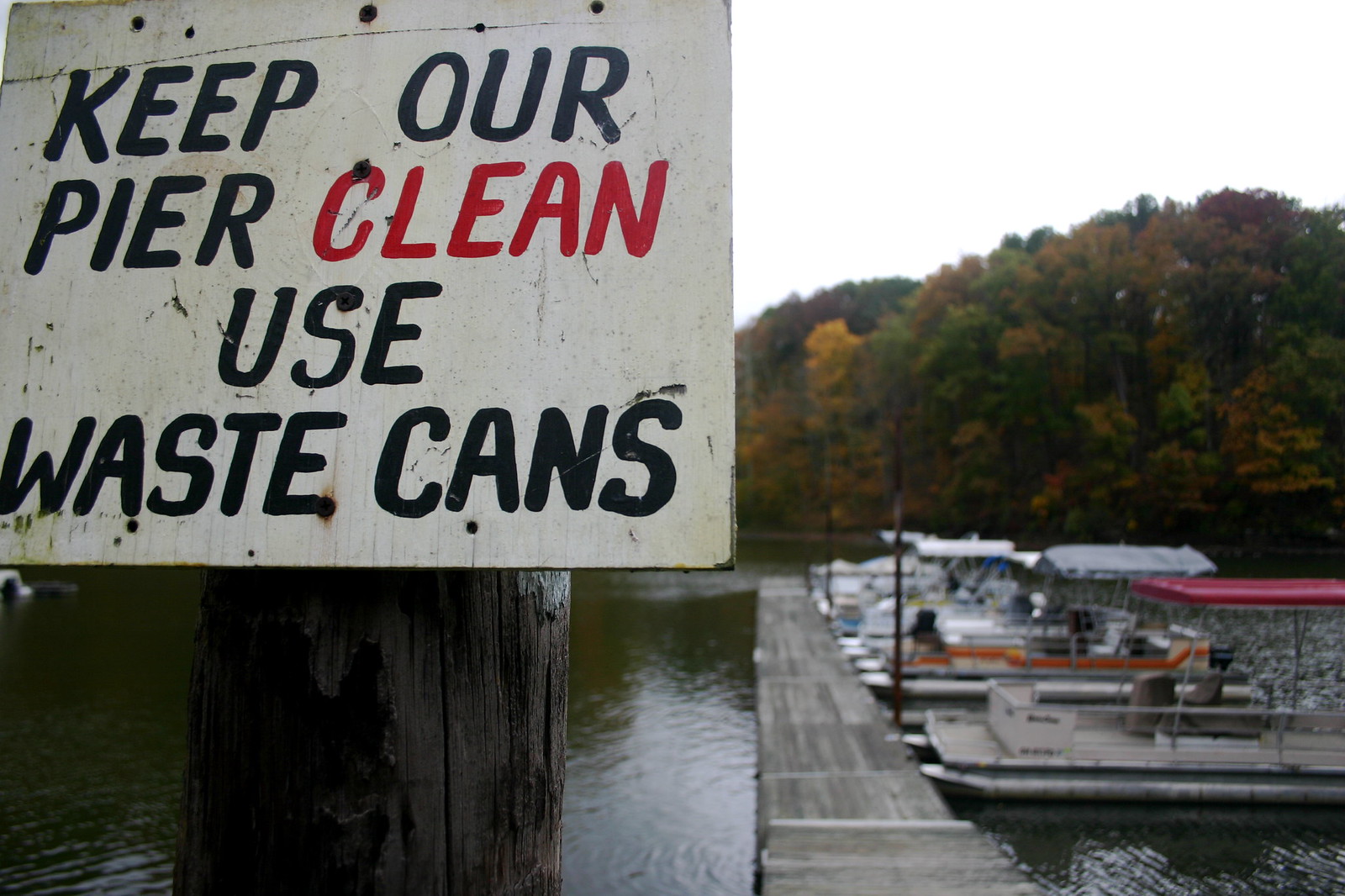The image depicts a busy dock scene on a lake during early fall. Dominating the left-hand side, a distinctive sign attached to a pier pole catches the eye, urging visitors with the message, “Keep our pier clean. Use waste cans,” where the word "clean" is emphasized in red, contrasting with the otherwise black text. The pier extends into the water, providing access to an array of boats docked on its left, including typical day boats and pontoon boats, one of which features a red canopy. The water has a notable greenish hue, reflecting the surrounding environment. Beyond the water, the background is adorned with vibrant fall foliage in hues of yellow, green, and rust-colored orange. The dock itself sports a gray surface, with boats neatly secured in their slips, against the backdrop of seasonally changing trees.